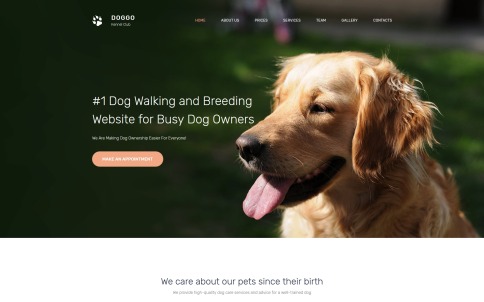The image depicts a website dedicated to pet services, prominently named "Doggo." In the top left corner, there is a logo featuring a paw print accompanied by the text "Doggo." The navigation menu to the right includes sections such as Home, About Us, Gallery, and Contacts, though some sections are difficult to read due to small font size. The main wallpaper of the site showcases a joyful golden retriever with its tongue playfully hanging out. Adjacent to the dog image, a headline reads: "Number One Dog Walking and Breeding Website for Busy Dog Owners." Below this, the text promotes the service with the statement: "We are making dog ownership easier for everyone." A clickable tab beneath the text invites users to make an appointment. At the very bottom of the page, a message underscores the company's dedication: "We care about our pets since their birth."